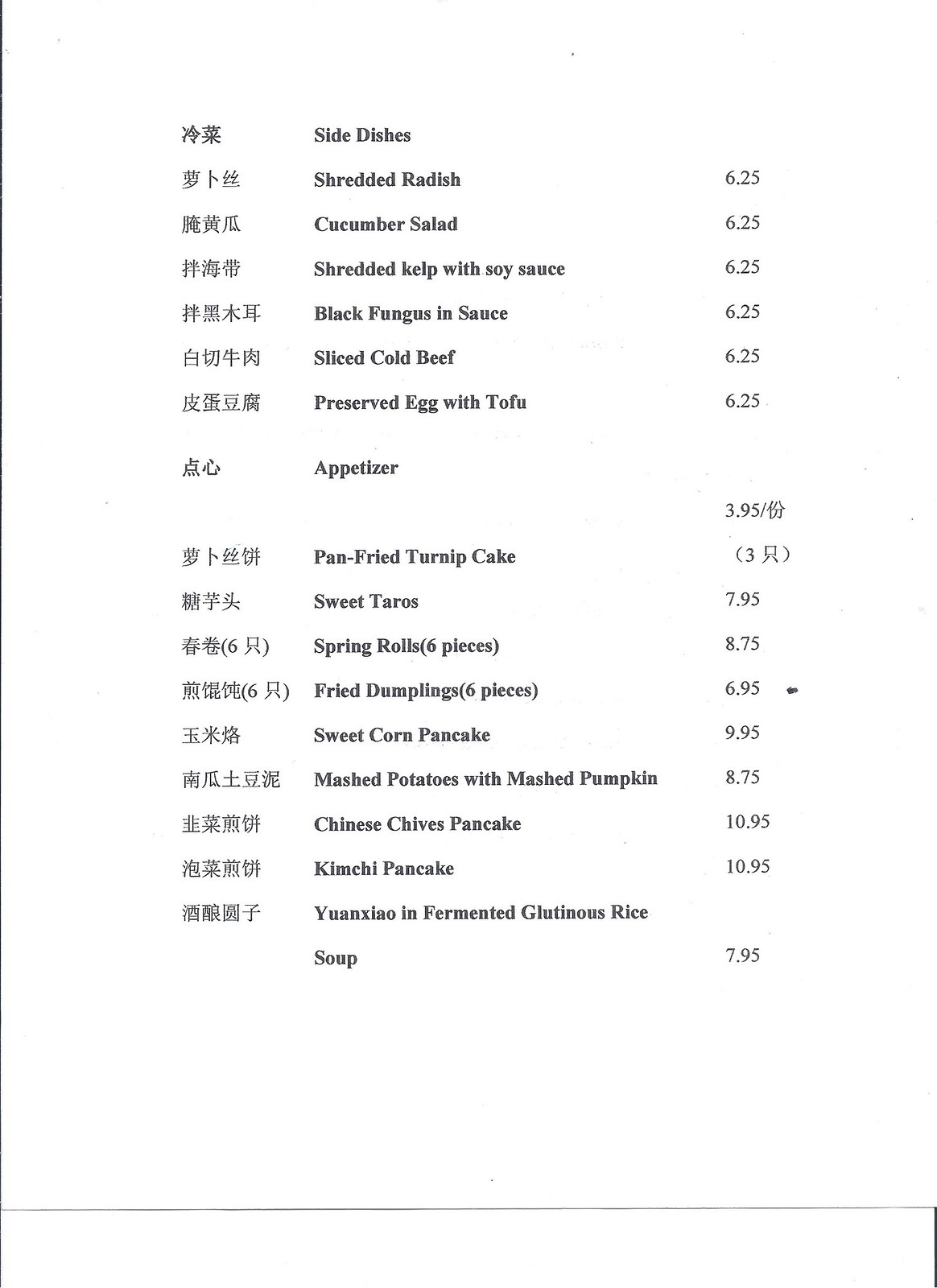The image displays a detailed menu highlighting various side dishes and appetizers, accompanied by their prices. The side dishes listed are: 

- Shredded Radish
- Cucumber Salad
- Shredded Kelp with Soy Sauce
- Black Fungus with Sauce
- Sliced Cold Beef
- Preserved Egg with Tofu

Each of these side dishes is priced at $6.25.

In addition to the side dishes, the menu showcases a variety of appetizers, which include: 

- Pan-fried Turnip Cake
- Sweet Taros
- Spring Rolls (6 pieces)
- Fried Dumplings (6 pieces)
- Sweet Corn Pancake
- Mashed Potatoes with Mashed Pumpkin
- Chinese Chive Pancakes
- Kimchi Pancake
- Yanjiao in Fermented Glutinous Rice Soup

The corresponding prices for the appetizers are: $3.95, $7.95, $8.75, $6.95, $9.95, $8.75, $6.95, $9.95, $8.75, $10.95, $10.95, and $7.95 respectively.

The text on the left side of the menu appears to be in either Chinese or Japanese, printed on a white paper background.